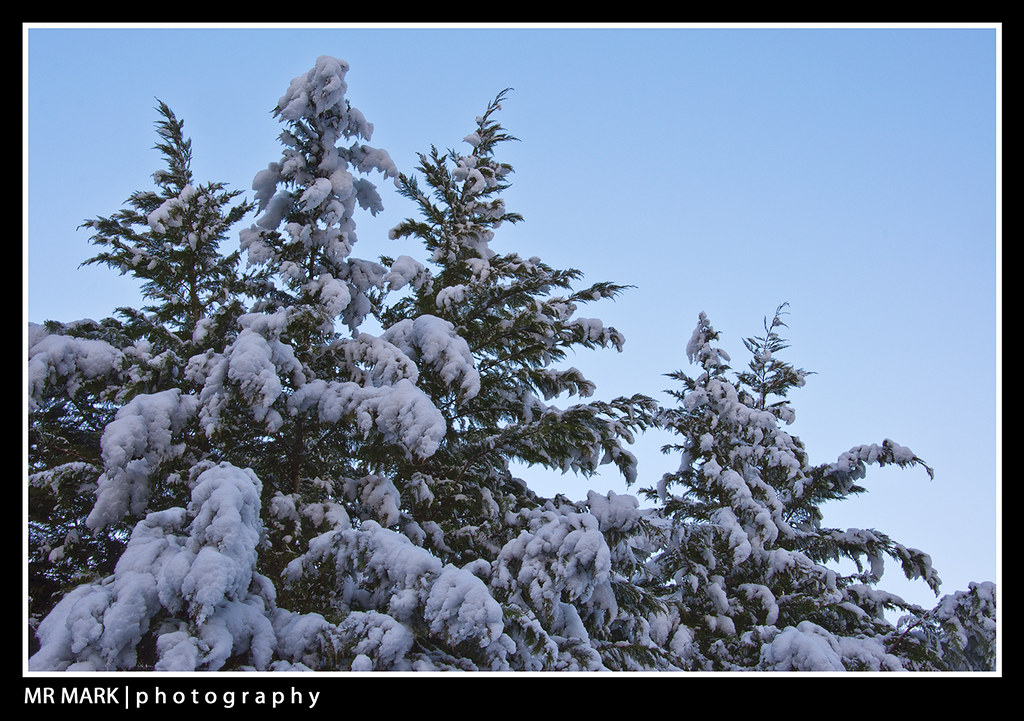This image, attributed to Mr. Mark Photography, captures a serene winter scene featuring snow-covered evergreen treetops under a clear blue sky. The evergreens, heavily laden with thick snow, dominate the foreground, creating a picturesque and tranquil winter landscape. The background reveals a gradient sky, transitioning from a light blue at the horizon to a deeper blue higher up, accentuating the crispness of the winter day. The photograph's quality and composition suggest a professional touch, even though opinions on the photographer's status vary. The image’s border is outlined in black with an inner white trim, giving it a postcard-like appearance. Notably, the photographer’s watermark, "Mr. Mark Photography," is subtly inscribed at the bottom, signifying the creator's pride in their work.